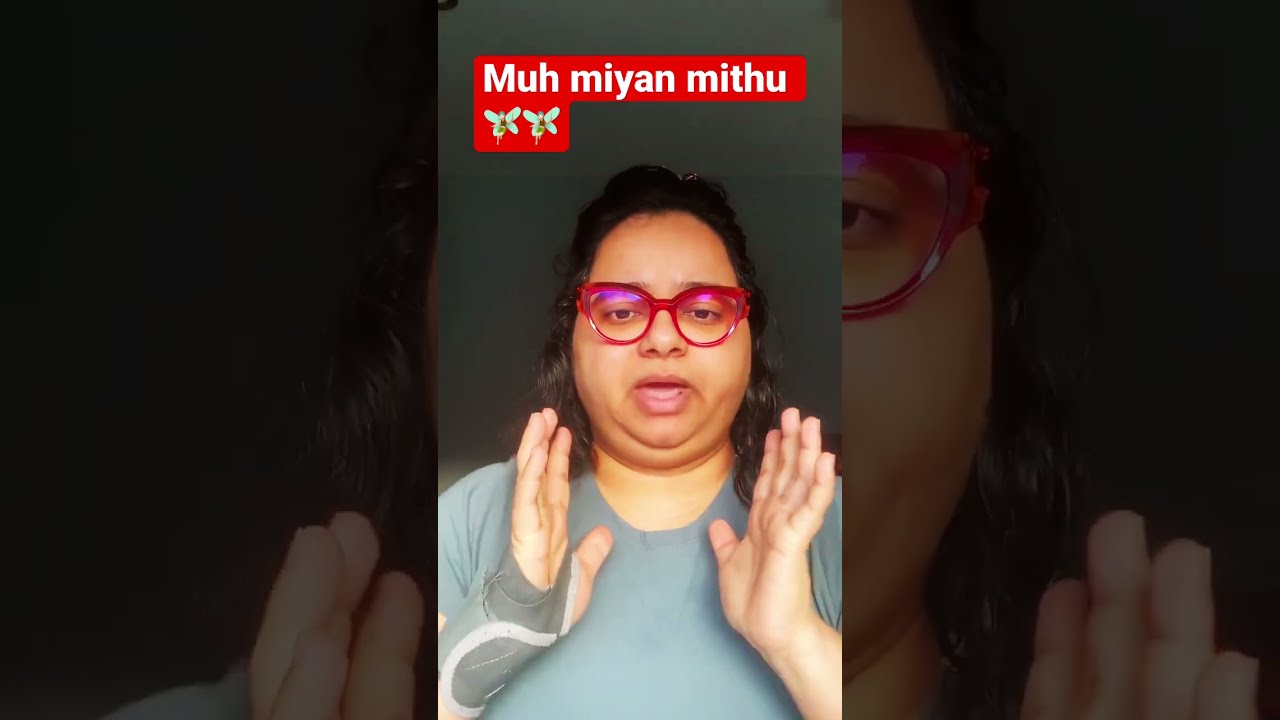This is a detailed photograph of an Indian woman with dark features, including black hair and brown skin, who is talking directly to the camera. She is slightly plump and has hot pink/red framed glasses. She is wearing a grayish-blue shirt and has a wrist brace on her right hand. The woman’s head is positioned in a way that creates a double chin, and she holds her hands in front of her chest with her palms facing each other as if explaining something. Her mouth is open mid-speech, possibly indicating surprise or deep engagement in her conversation.

The background is a grayish-black, making it hard to discern further details. Above her head, there is a red text box with white lettering that reads "MUH MIYAN MITHU" (or "Mua Mian Mitu"), and below the text are two butterfly/fairy emojis. This main image is bordered on the left and right sides with zoomed and darkened portions of the same image to create a seamless frame.